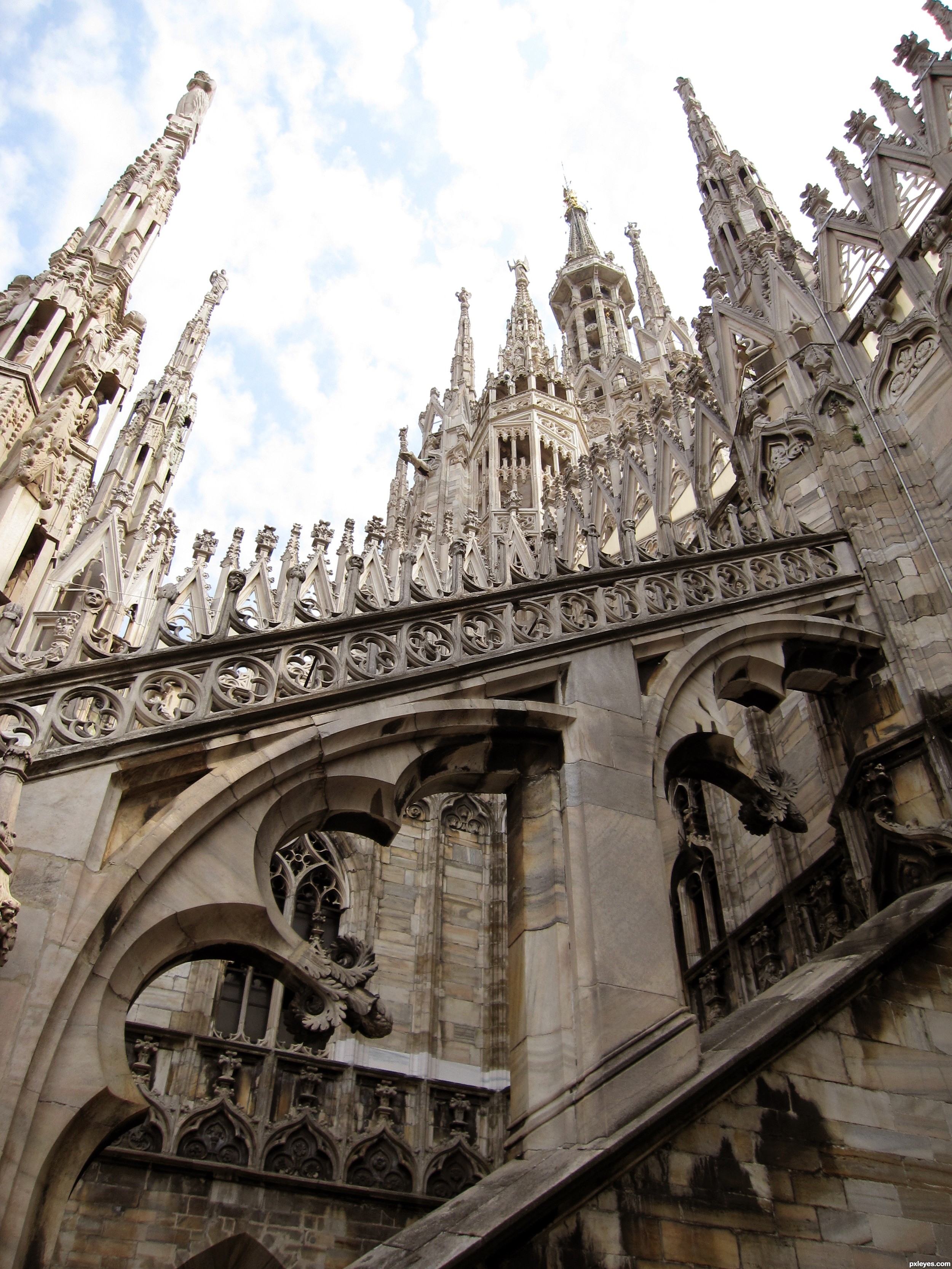The photo captures a stunning, ancient Catholic cathedral with a Gothic architectural style, characterized by its ornate and intricately decorated spires. Taken from a dramatic upward angle, the image showcases numerous spires that reach towards the sky, adorned with small columns and statues that appear to be angels. The structure, built from large beige and brown stones, exudes a sense of history and timelessness, reflecting the craftsmanship and detailed construction typical of such venerable churches. While the full view of the cathedral is not visible, the elaborate spires and church crosses lend a sense of grandeur and reverence to the scene.